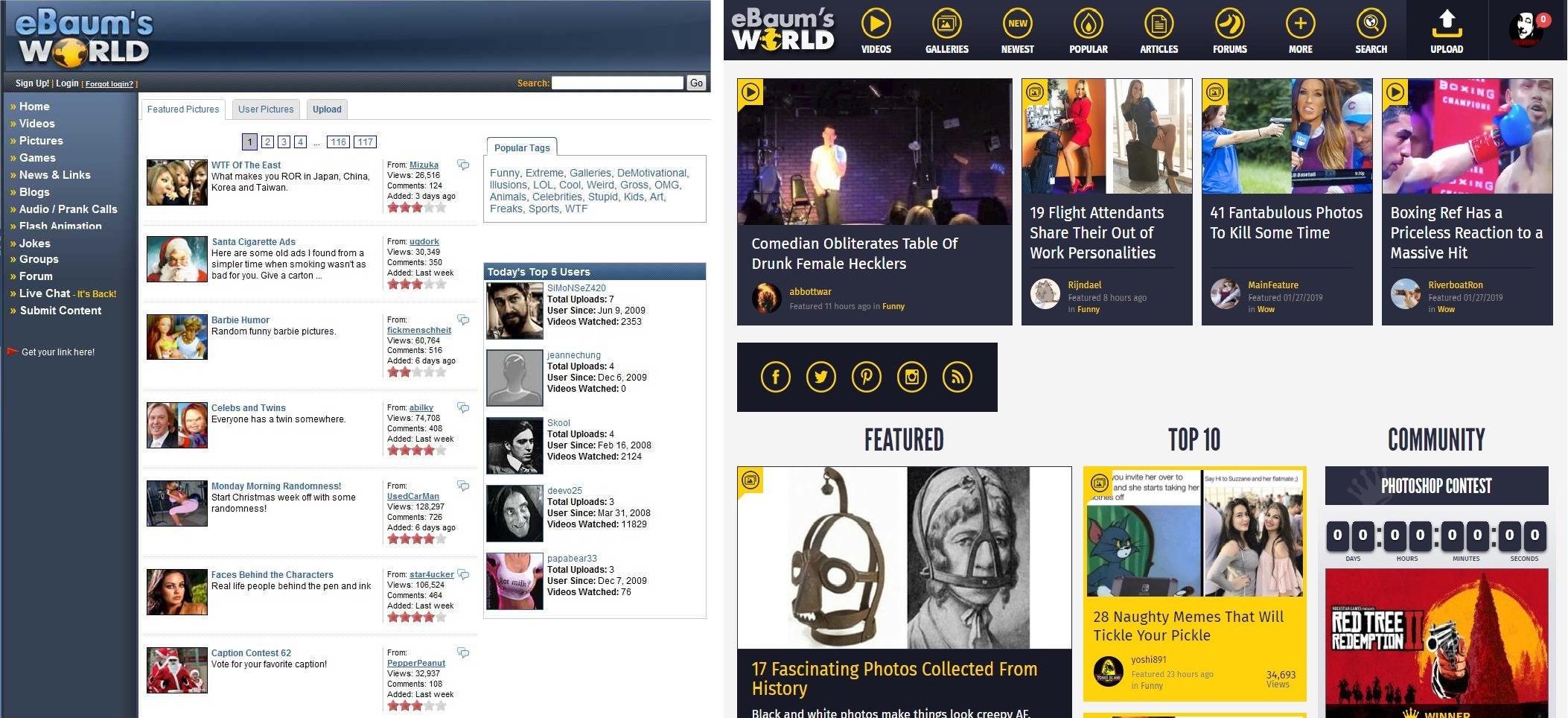The description provided details a side-by-side comparison of two images. Here is a cleaned-up and detailed caption:

---

**Side-by-Side Comparison of Two Images:**

**Left Image:**
- **Background Gradient:** The background transitions from dark blue at the top to a lighter blue towards the bottom.
- **Header:** "eBombs World" is prominently displayed at the top.
- **Menu Bar:** Below the header, there is a menu featuring white text. 
- **Content Section:** A large white square dominates the center of the image.
  - **Left Side of the Square:** A vertical row of pictures.
  - **Right Side of the Pictures:** Descriptive text in alternating blue and black fonts.
  - **Ratings:** Positioned to the right of the text, represented by stars.
    - **First and Second Text Sections:** 3 stars each.
    - **Third Text Section:** 2 stars.
    - **Fourth to Sixth Text Sections:** 4 stars each.
    - **Seventh Text Section:** 3 stars.
- **Additional Images and Text:**
  - **Below the initial row:** Five more pictures displaying individual portraits.
    - **Subjects:** Men and women, including a woman in a white tank top with noticeable features.
    - **Text:** Blue text beneath each picture, with additional black text below.
- **Top Left Corner:**
  - **Search Bar:** White search bar with the word "Search" in gold letters.
  - **Gray Button:** Positioned to the right of the search bar.

**Right Image:**
- **Subjects:** Several individuals depicted in different poses.
  - **Examples:** A boxer and a person on stage.
- **Background:** Plain white, making the subjects stand out.

---

This caption provides a thorough and detailed description of both images, enhancing visual comprehension for the reader.